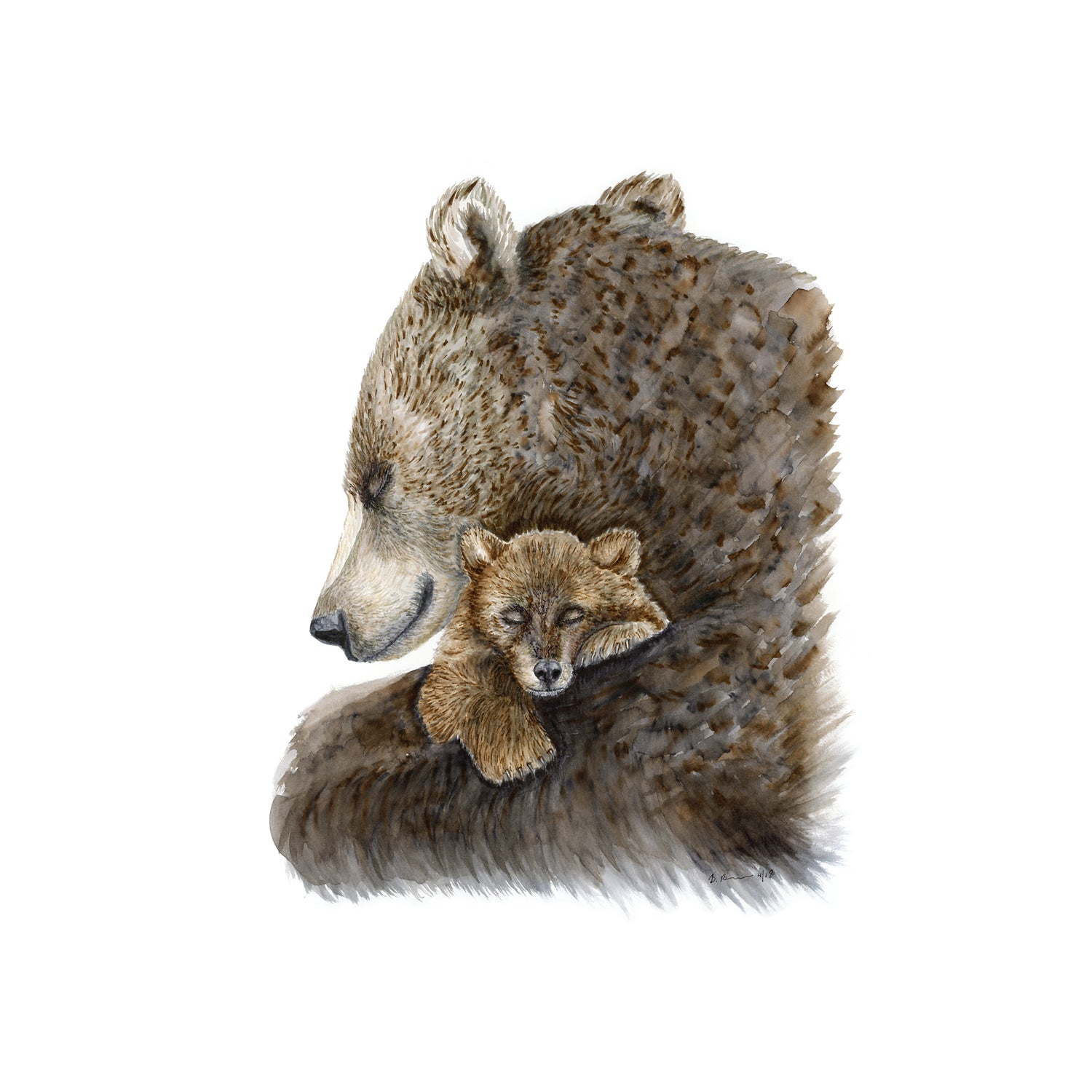In this watercolor-like painting, we see the gentle embrace of a mother grizzly bear cradling her cub under its chin with its front legs. The maternal bear, facing left, displays a spectrum of colors from a very white face, light brown around the top of its face and ears, to dark brown and light gray in its body which gradually dissolve into less intricate blobs. Her eyes are closed, and she wears a serene smile. The cub, golden in color with a little white on its face, also has its eyes shut, adding to the tranquil ambiance of the scene. Only the head and the front legs of the cub are visible, nestled securely under the mother's chin. The right edge of the painting cuts off just where the mother bear's neck would be, focusing our view on this intimate moment between the mother bear and her cub.